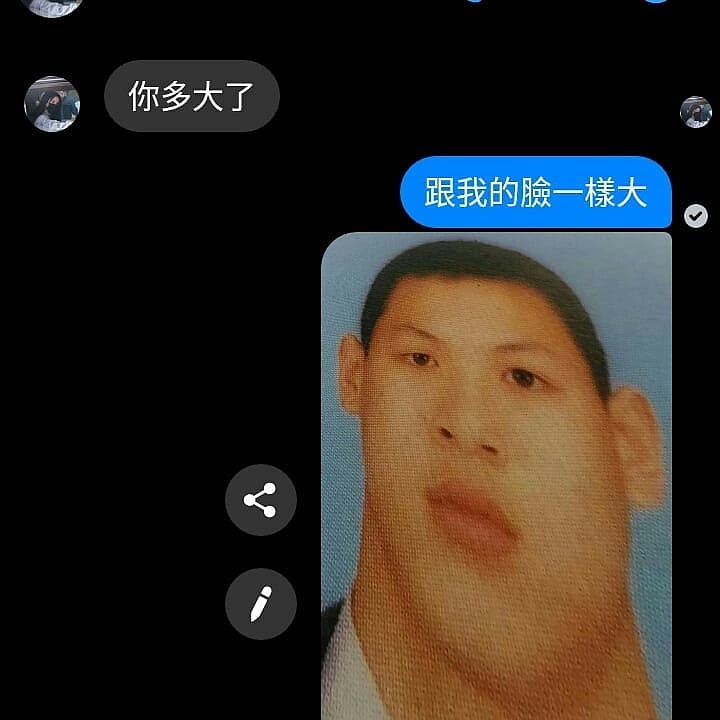The image is a digital screenshot, likely taken from an iPhone or Android device, showcasing a conversation between two individuals in a non-English language, possibly Chinese or Korean. The central element of the screenshot is the photograph of a young Asian man in his 20s with black hair and black eyes. His face, unusually elongated, appears to be edited, possibly for comedic effect. Text, possibly indicating the name 'Renaleigh,' is displayed in blue immediately above his photograph. Additional text appears on the left side against a gray background. The conversation, indicated by the foreign script, suggests a personal interaction, potentially humorous, as suggested by the unusual alteration of the man's photo. The entire screenshot background is black, hinting that the image might be from iMessage or a similar messaging app, which also allows further sharing or editing options.